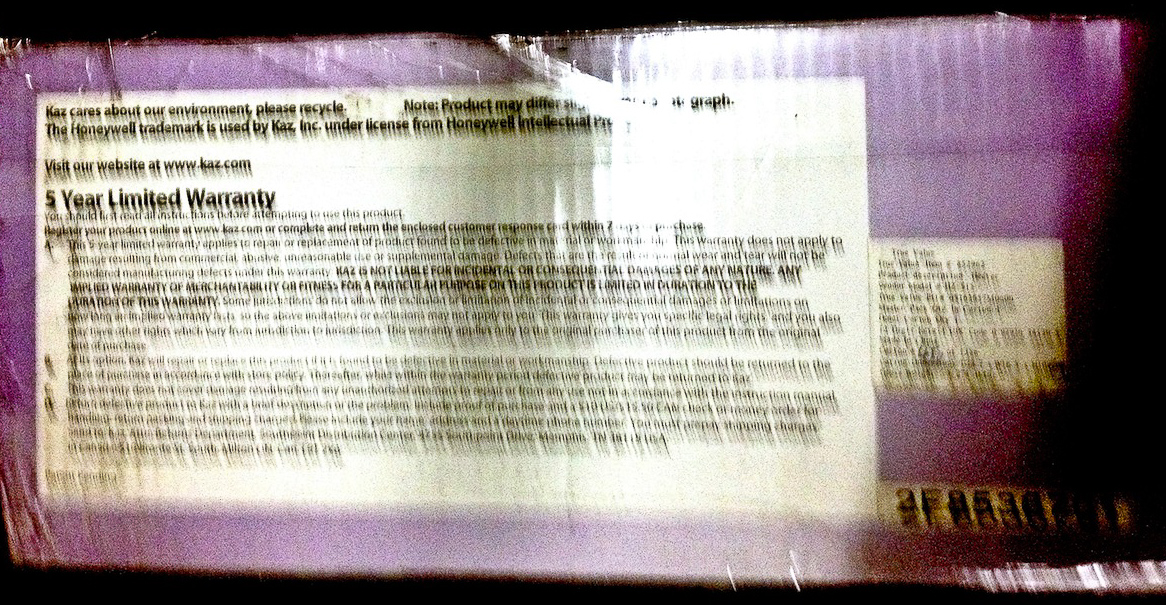This horizontally rectangular image features a blurred scene with thin black borders running horizontally along the top and bottom edges and a vertical black border on the right side. At the center, a purple corrugated box is visible, with the texture accentuated by a noticeable glare. Resting on the box's surface is a white, horizontally oriented rectangular label. While most of the text is illegible, the label prominently displays "5-year limited warranty," accompanied by smaller, unreadable verbiage. The overall image quality and glare obscure further details, but the box's corrugated texture remains discernible.